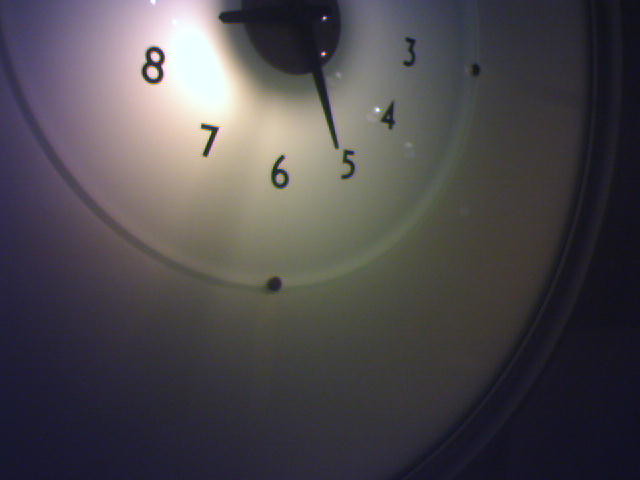This close-up photo captures a white clock, emphasizing a segment of its face that displays the numbers three through eight. The clock features a concentric design, with a darker outer circle framing a lighter inner circle. Black clock hands extend outward from a small dark center. Notably, there's a reflection between the numbers seven and eight, hinting at a light source shining on the clock. The lower right-hand corner of the image fades into a dark background, creating a stark contrast that highlights the illuminated portion of the clock.